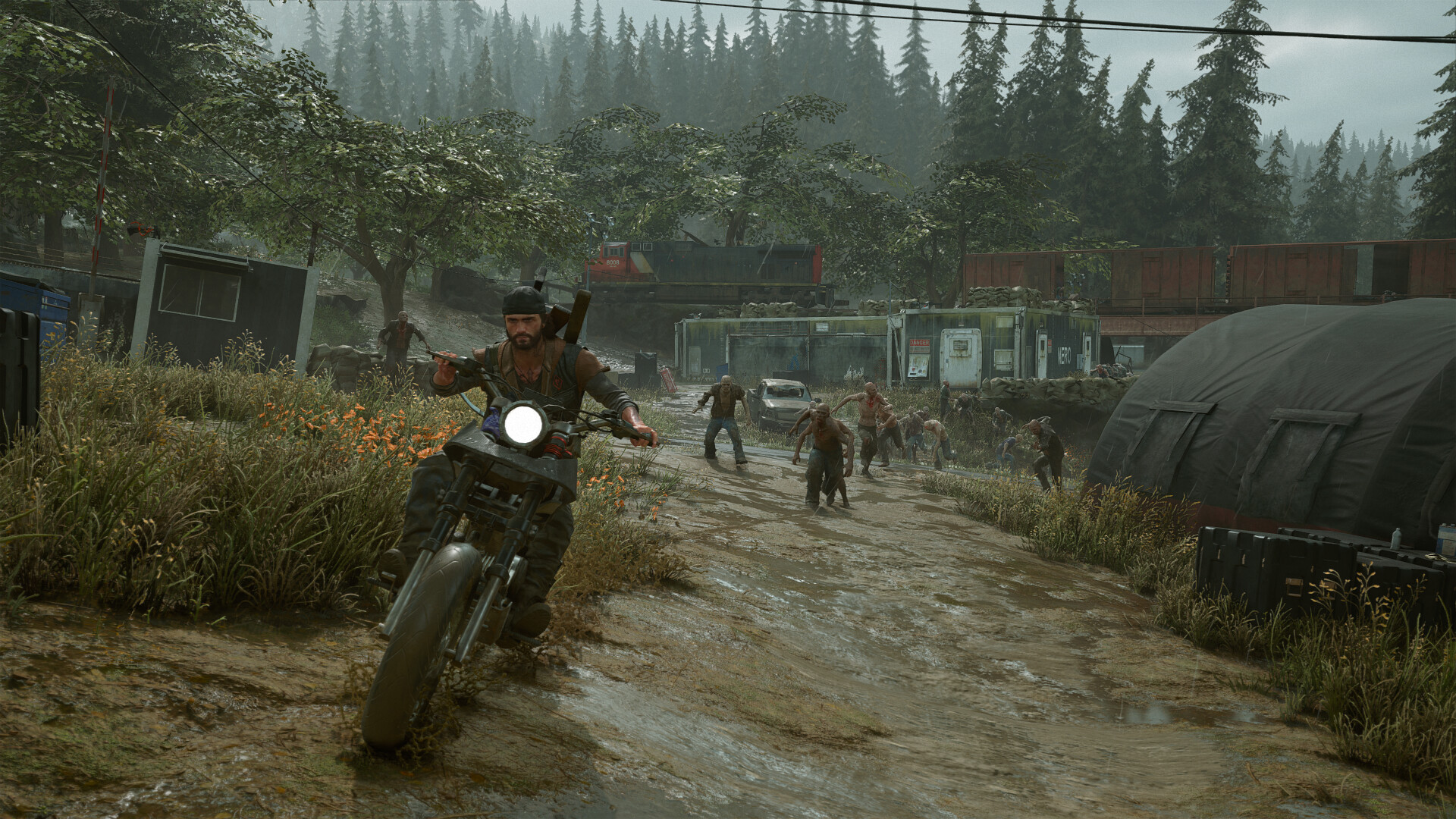The image appears to be a dynamic scene, likely from a video game, depicting a tense moment in a wet, muddy forest area, possibly during or after a rain. At the forefront, a man with a military-style bandana or cap is riding a motorcycle directly towards the viewer. The bright, circular white headlight of the motorcycle is distinctly visible. The motorcyclist navigates a muddy dirt road flanked by vegetation and colorful orange flowers. Surrounding the area are elements indicating a makeshift encampment; to the right sits a military-style greenhouse structure with fabric tarps, accompanied by storage containers. In the midground, several disheveled, shirtless men, possibly zombies due to their aggressive demeanor, chase the motorcyclist. The background showcases tall pine trees, a fenced area surrounding dumpsters, and a passing train with container-like buildings scattered nearby. The scene exudes a post-apocalyptic military vibe, complete with the chaos and urgency typical of survival scenarios.